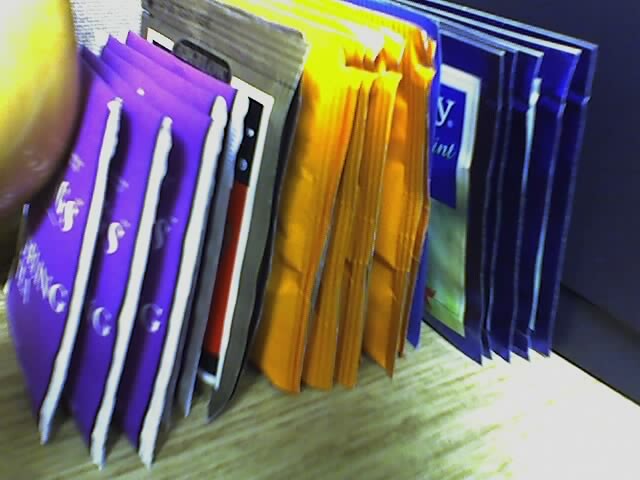The image showcases an assortment of tea packets and a banana on a wooden shelf, taken with flash in a dim environment, illuminating parts of the scene. The tea packets are leaning against each other towards the right. Starting from the left, there is a yellow banana adjacent to four square blue packets, likely Twinning's tea. Following the blue packets, there’s a noticeable silver packet, then several yellow tea bags, possibly Bigelow teas. On the far right, there is another blue packet, and five more dark blue packets featuring white text framed in blue squares. The packets are neatly arranged in a row like files, set against a dark blue background with pale white highlights. The lower right corner of the image is brightly illuminated, possibly by the camera flash.